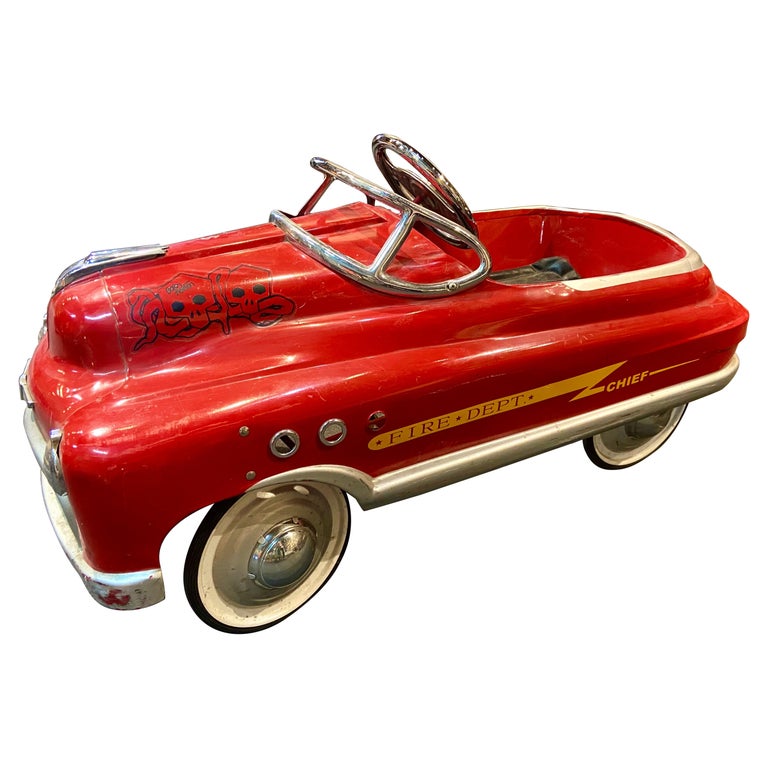This horizontal photograph captures a nostalgic red toy car designed for young children to ride in, reminiscent of an old-fashioned convertible from the 1940s or 1950s. The car's body is crafted from metal, decorated with a yellow lightning bolt and the words "fire department" on one side and "chief" on the other. The car narrows toward the back and features a raised center from the steering wheel to the front, imitating a vintage engine hood. 

It stands on thin black tires with white walls and gray hubcaps, resembling those of a little red wagon, and is accented by a chrome bumper and a silver trim along the bottom. A distinctive silver hood ornament graces the front, and a decal with two skulls and a snake adds a touch of rugged flair to the hood. The steering wheel, rising above the windshield frame—a simple, glassless piece of silver metal—suggests a playful, imaginative experience for a child. An inviting seat behind the steering wheel indicates where a child could sit, placing their feet on the ground to propel the car, as there are no pedals included. This charming toy car sits against a clean white background, emphasizing its detailed, classic design and inviting viewers to reminisce about a bygone era of childhood play.